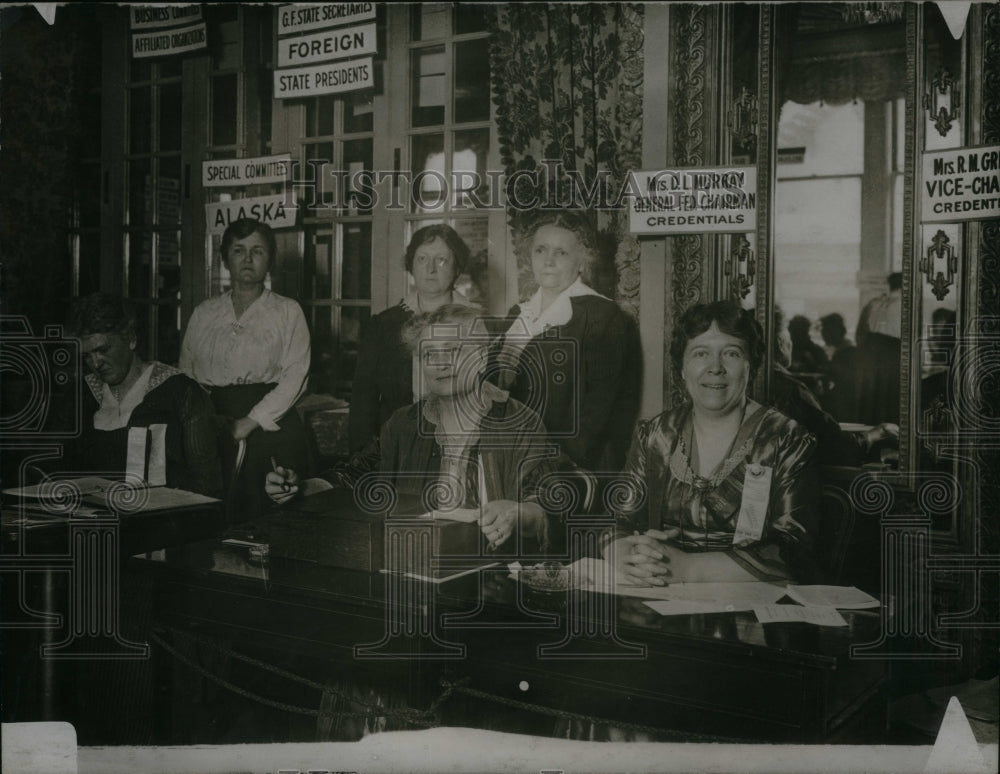This historic black-and-white photograph captures a group of six women in what appears to be an official, possibly electoral setting. The image is faint and obscured by watermarks reading "Historic Image" and symbols resembling a camera and a podium. In the forefront, three women are seated at a long, shiny wooden table cluttered with papers and miscellaneous items. 

Starting on the left, the first woman has short hair and is adorned with a white lacy piece around her neck and shoulders, over a darker garment. She looks down to her left. Directly behind her stands a woman with short, dark hair, a white shirt, and a dark skirt, gazing straight ahead. Beside her, another standing woman with short curly hair and glasses wears a dark coat and looks slightly to the left.

At the table, parallel to the aforementioned trio, another seated woman with short grayish hair and a dark coat looks forward and slightly to the left. Behind her stands a woman turned a bit to the left, dressed in a white shirt and dark coat, with blonde hair reaching her shoulders or just below her ears, wearing a hat. 

The last woman, on the right side of the image, sports a blouse with dark and light patterns and has short, dark, curly hair. She faces straight ahead, and on the table before her are scattered papers. The backdrop includes large white door frames with window panes, reflecting a somewhat professional, perhaps governmental environment, possibly from the 1960s. Signs in the background hint at the context of the setting, with phrases like "GF State Secretaries," "Foreign State Presidents," "Special Committee," and "Alaska," suggesting these women might be involved in state election processes or official record-keeping.